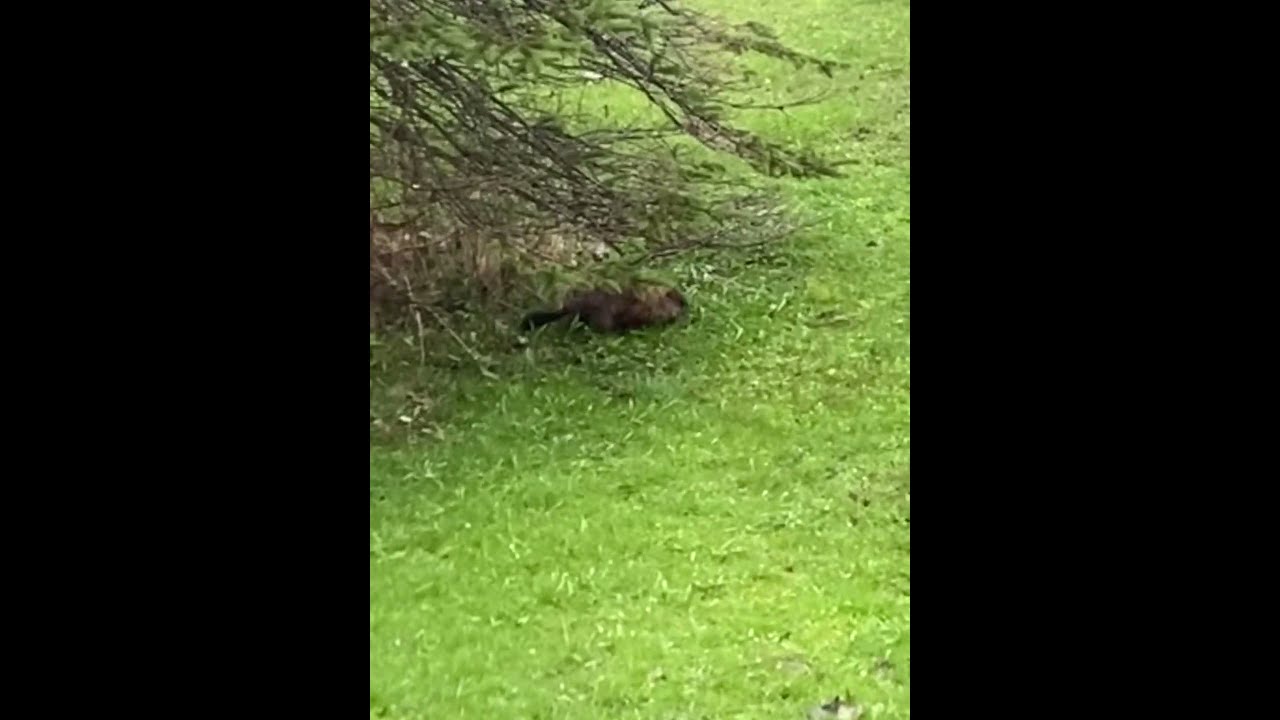This horizontally aligned photograph with thick black borders framing a narrower rectangular image captures an outdoor scene during the daytime. The main focus is a small, brown animal occupying the center of the lush, green grassy field, which has occasional patches of dead, tan grass. The animal appears to be a rabbit, identifiable by its brown fur and ears down as it eats something, although the image is somewhat blurry, leading to some uncertainty about its exact species.

Above the rabbit, extending from the upper left corner and reaching down towards the ground, are a mix of live and dead tree branches. These branches, some adorned with green leaves or pine needles and others barren, add a textured canopy over the grassy area. Toward the top right corner of the photograph, the terrain seems to incline, suggesting a hill. The overall composition captures the interplay between the verdant and dry elements of the landscape, framing the rabbit in its natural, yet slightly barren habitat.